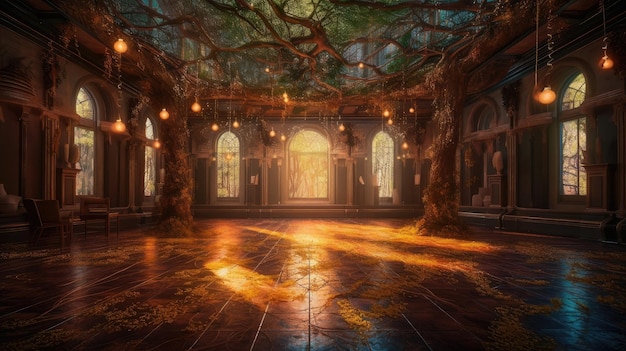The image captures an ornate, elegantly designed indoor space, possibly a painting or highly detailed photograph, that evokes a mystical and almost cinematic atmosphere. The room features seven large, arched windows through which rays of light pour in, creating a warm, golden essence on the brown, wooden plank floors. There are two prominent indoor trees positioned on either side of the room, their limbs stretching towards the ceiling and adorned with low-hanging orange lights that resemble ornaments. The bloom effect of the light enhances the enchanting ambiance, making the space feel like a serene yet otherworldly abode, reminiscent of a place where a witch might live. The intricate roof and walls add to the luxurious aesthetic, with a mix of brown and green tones from the ceiling foliage, contributing to the room's overall splendid and elegant allure.